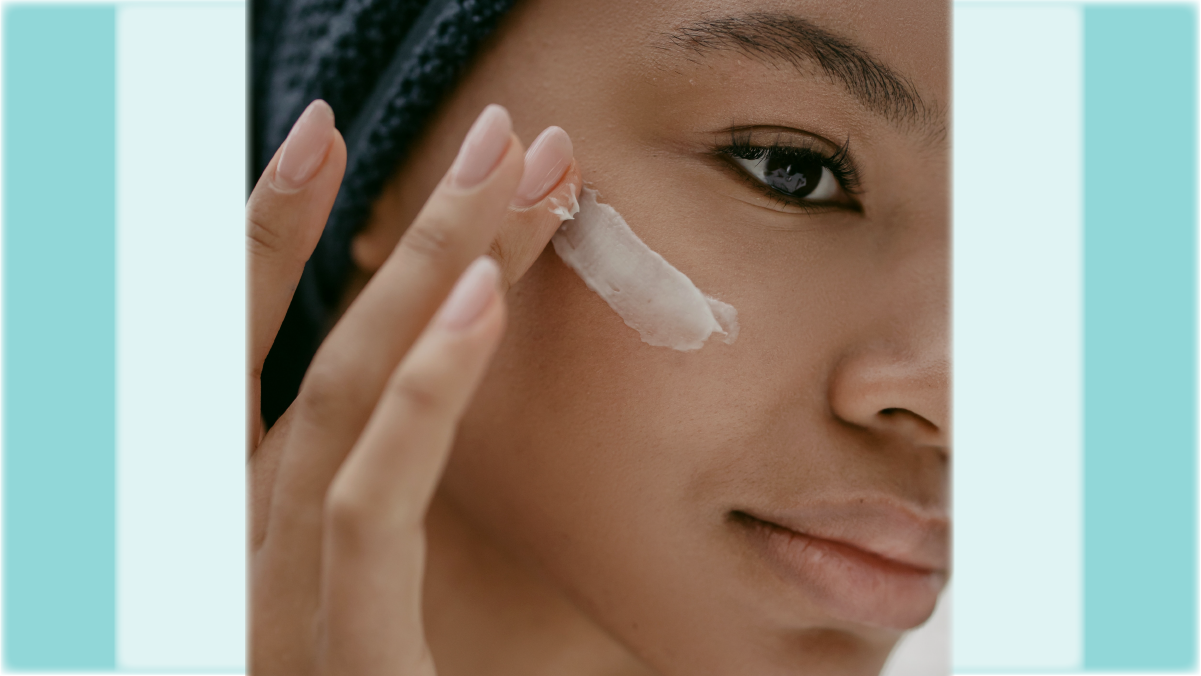In this image, a person with medium-dark skin is applying a white skin cream to their cheekbone area using their middle finger. Their face is partially turned at a diagonal to the right, revealing only one brown eye, half of their nostril, and most of their lips. Subtle dark eye makeup enhances their visible eye, and their nails are painted a very light pink. Their black hair is styled in braids, visible towards the upper left of the image. The cream is being applied with their fingers, which are positioned on the side of their face. The image has multiple borders: a thick light blue one around the main image, followed by a slightly darker blue border on the left side, and another on the right side.